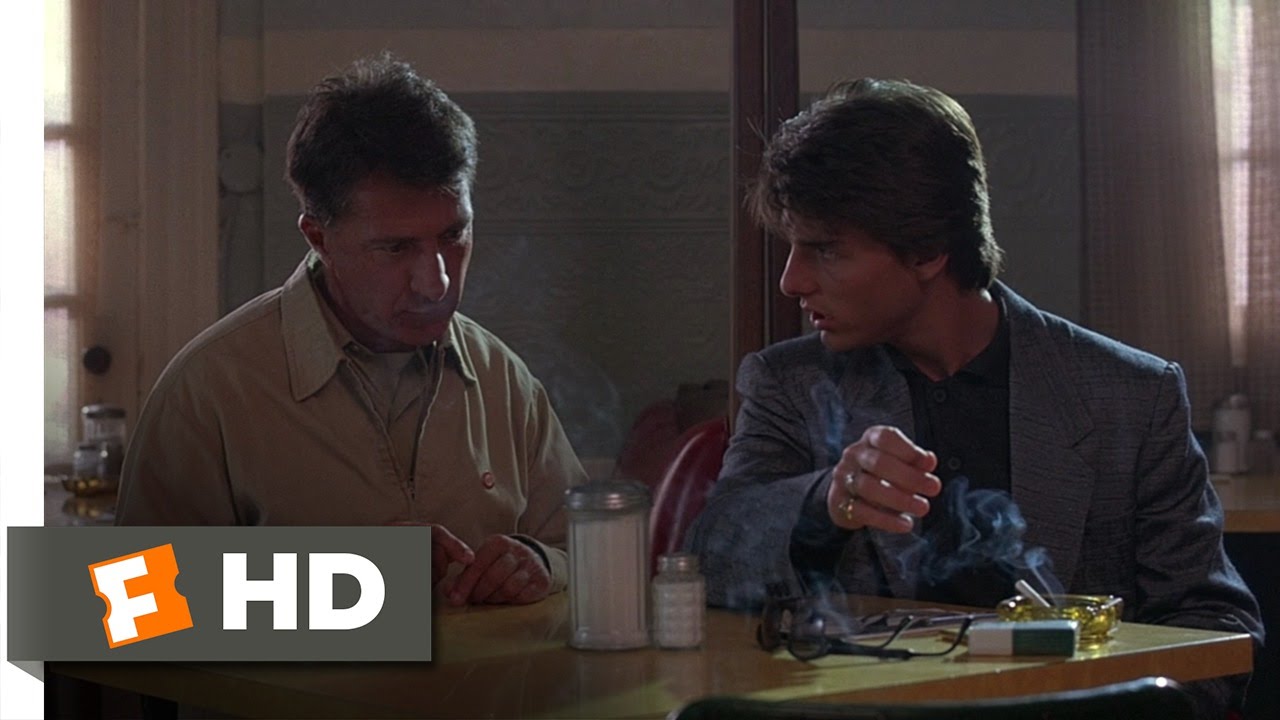This detailed screenshot from the movie "Rain Man" captures a scene featuring Tom Cruise on the right and Dustin Hoffman on the left. Both actors are seated at a wooden table. Tom Cruise, dressed in a grayish suit with a black shirt beneath, looks to the left, directing his gaze at Dustin Hoffman, who is wearing a tan jacket and appears to be staring at the table's contents. The table holds a smoldering cigarette in an ashtray, a cigarette box, a pair of sunglasses, as well as a salt and sugar shaker. In the background, there's a gray wall with a white upper portion, along with curtains and a window on the right, and a white door to the left. On the bottom left corner of the video clip, there's a small Fandango logo resembling an 'F' inside a ticket, followed by the label 'HD' in white.